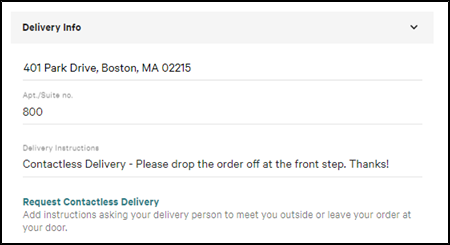A screenshot with a white background displays a gray rectangle containing delivery information in black text. The information includes a down arrow followed by the address "401 Park Drive, Boston MA 02215." It also specifies an apartment/suite number with "apt. and number," though the details are labeled as "nl." Additionally, the number "800" is displayed.

The screenshot highlights delivery instructions requesting contactless delivery with the note: "Please drop the order off at the front step, thanks." There is also a blue link labeled "Request contactless delivery," which allows the user to add further instructions, asking the delivery person to either meet them outside or leave the order at the door.